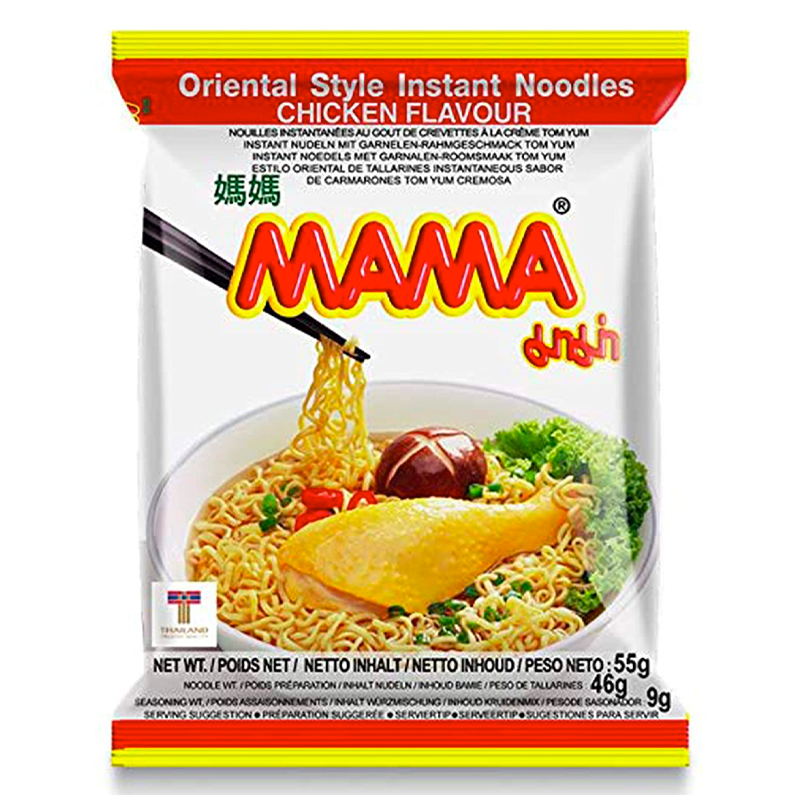This detailed close-up photo depicts a packet of Oriental style instant noodles, specifically chicken flavor. The packaging features a predominantly white background with vibrant orange and yellow strips running along the top and bottom edges. Dominating the center is an enticing image of a white bowl brimming with noodles. A succulent chicken drumstick rests atop the noodles, complemented by an array of vegetables including greenery and broccoli. To the right of the chicken, there's a split-open potato. Above this appetizing scene, a pair of chopsticks lifts a mouthful of noodles from the bowl. Prominently displayed above the bowl, in large red capital letters with a yellow border, is the brand name "Mama." The packaging also includes text in French at the top, which reads "Oriental style instant noodles, chicken flavor" in white font. Scattered around the package are additional characters, likely in Chinese or Japanese, providing further details. The net weight of the contents is listed in four different languages at the bottom.